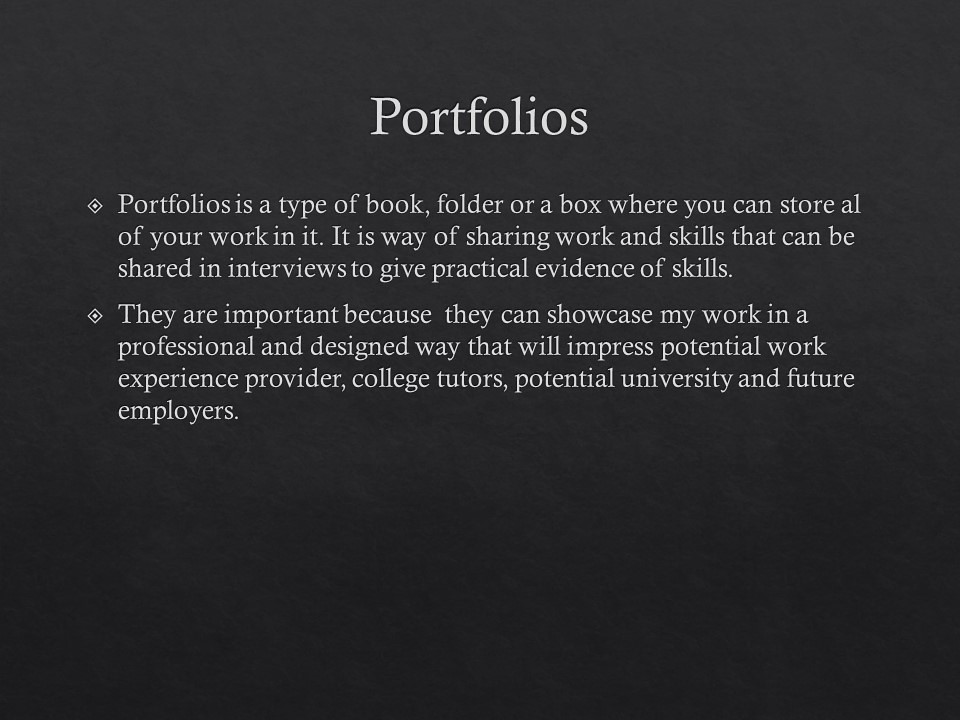The image depicts a single slide from a horizontally oriented PowerPoint presentation. The slide has a dark, blurred gray or black background. At the very top, centered, is the title "Portfolios" in white text. Below the title are two bullet points, each marked with a diamond-shaped bullet rather than a traditional circular one. The first bullet point reads: "Portfolios is a type of book, folder, or a box where you can store all of your work in it. It is a way of sharing work and skills that can be shared in interviews to give practical evidence of skills." The second bullet point states: "They are important because they can showcase my work in a professional and designed way that can impress potential work experience providers, college tutors, potential universities, and future employers."